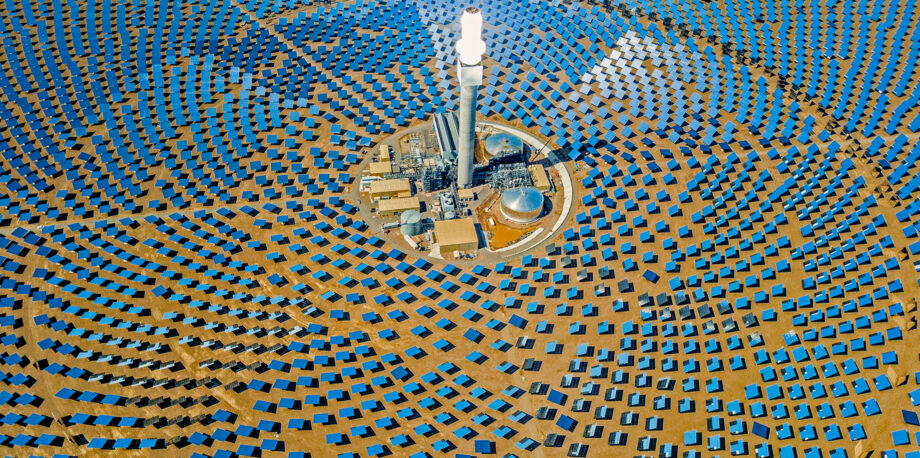In the image, a circular structure stands isolated amidst a barren, dirt-covered expanse, devoid of trees or any signs of civilization. At the center of this structure, a tall pole with a light extends upwards, surrounded by an array of blue panels. These panels, likely solar in nature, are arranged in concentric circles around the pole, suggesting that this installation harnesses solar power. The overall setup hints at a solar power plant, rather than an amusement park, given the absence of recreational elements and the functional, energy-focused design.